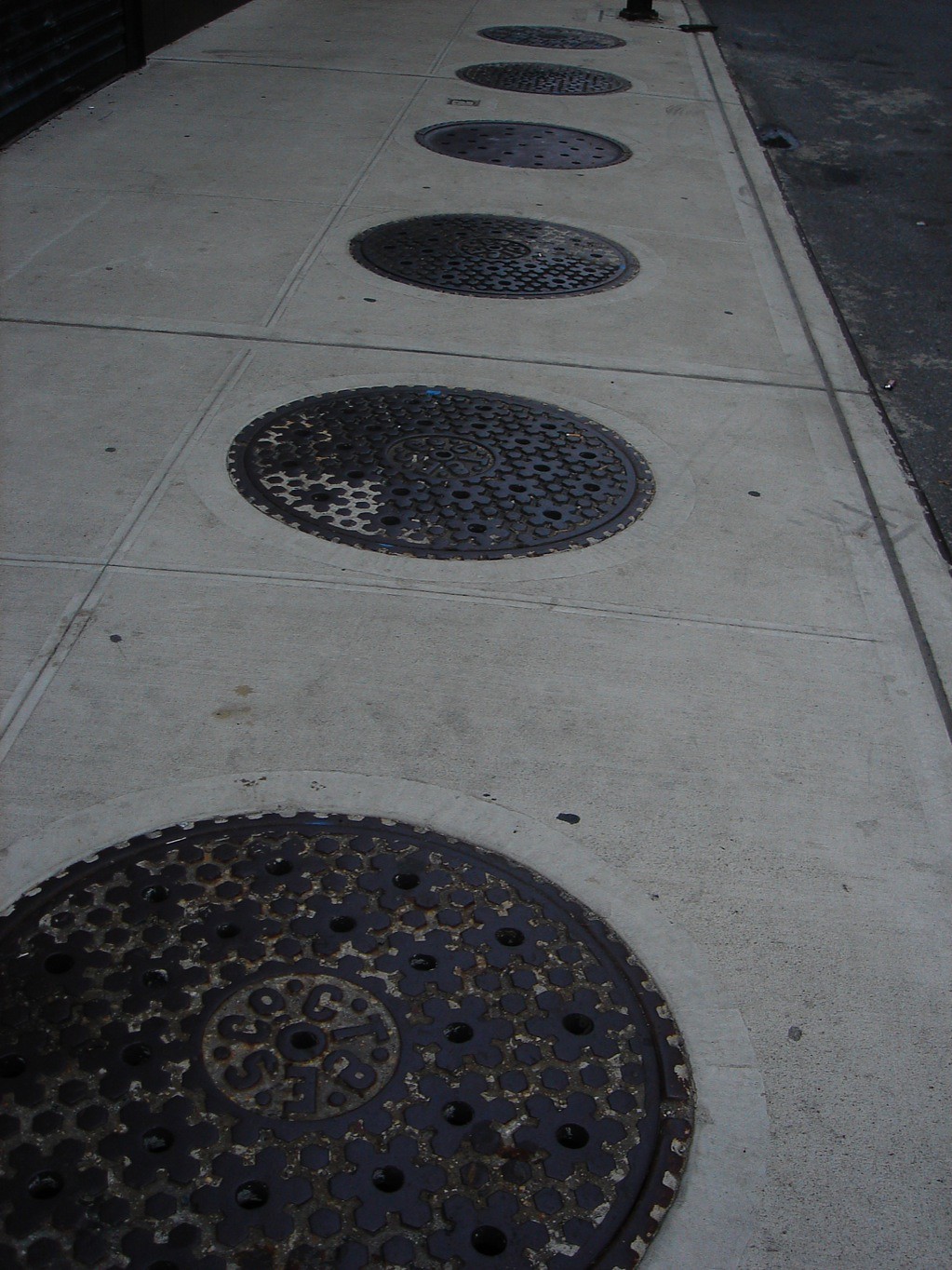This black-and-white photograph captures a wide section of a street or sidewalk, primarily composed of light gray pavement. The dominant feature in the image is a row of six rusted cast-iron manhole covers, positioned in a straight line stretching from the bottom toward the top of the photo. Each manhole cover, approximately two to three feet in diameter and spaced about three feet apart, is adorned with intricate flower patterns and marked with multiple holes. Additionally, some covers display the letters "S-E-C-O." Surrounding the light gray central strip of pavement, darker asphalt from what appears to be a road edges the sides, adding contrast and emphasizing the orderly procession of manholes.